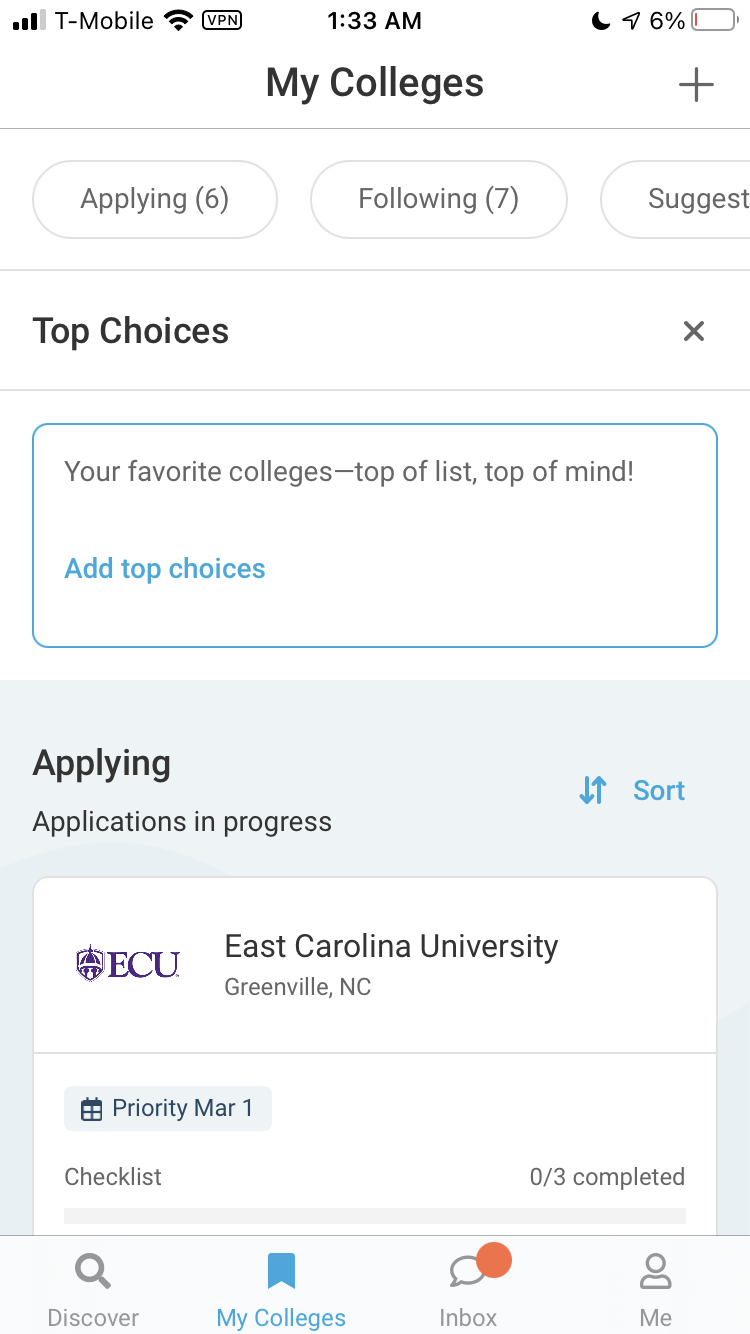In the image, a smartphone screen is displayed with the following details: At the top, the screen shows three bars for signal strength, a T-Mobile carrier label, a battery level at 6%, and the time as 1:33 a.m. The main content area highlights a section titled "My Colleges." The section contains an organized list, which starts with "Applying: 6" and "Following: 7." Below, a label says "Suggest" without any numbers provided.

The focus then shifts to a white rectangular box with a blue border, indicating "Your Favorite Colleges: Top of List, Top of Mind." A blue hyperlink labeled "Add Top Choices" is visible. Underneath this section is a light blue box that says "I'm Applying."

Directly below is another white box showing application progress details, marked "Application to Progress." There is a blue, up-and-down arrow hyperlink labeled "Sort." Inside this box, you see the ECU logo along with the text "East Carolina University, Greenville, North Carolina," and a priority deadline marked as "March 1st." Additionally, there is a checklist with the status "0 of 3 completed." At the bottom of the screen, you can see navigation labels: "Discover," "My Colleges," "Inbox," and "Me."